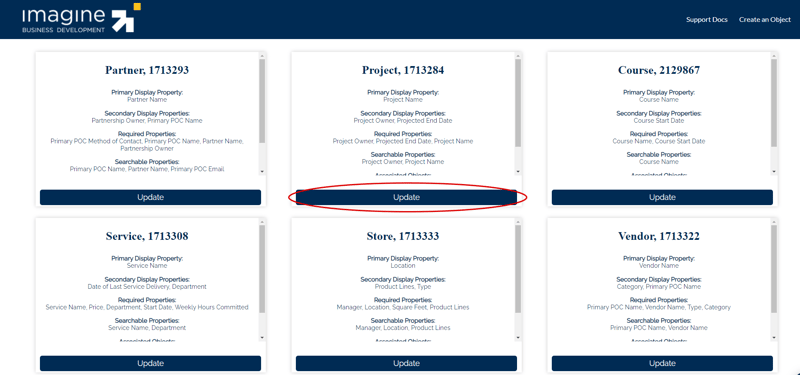This image features a designer promoting business development within a structured layout. The top section showcases a blue banner with text; "imagine" is in lowercase white letters, while "BUSINESS DEVELOPMENT" stands out in uppercase. An upward, pixelated arrow pointing to the right is positioned near a logo. 

The lower part of the image consists of a white background with a separated body and an orange, diamond-shaped tip. 

On the right side, the text reads "SUPPORT DOCKS OR CREATE AN OBJECT." Below this, there are six squares arranged in two rows of three. Each square contains different text: "PARTNER 17132993" presents primary display property as the partner name, alongside secondary, required, and searchable properties; the middle squares describe a project along with its number and display properties. Each square at the bottom has a blue bar labeled "UPDATE" in white.

Notably, the middle square is circled in red. The bottom row labels are "SERVICE," "STORE," and "VENDOR," each having the same detailed fields as the other squares.